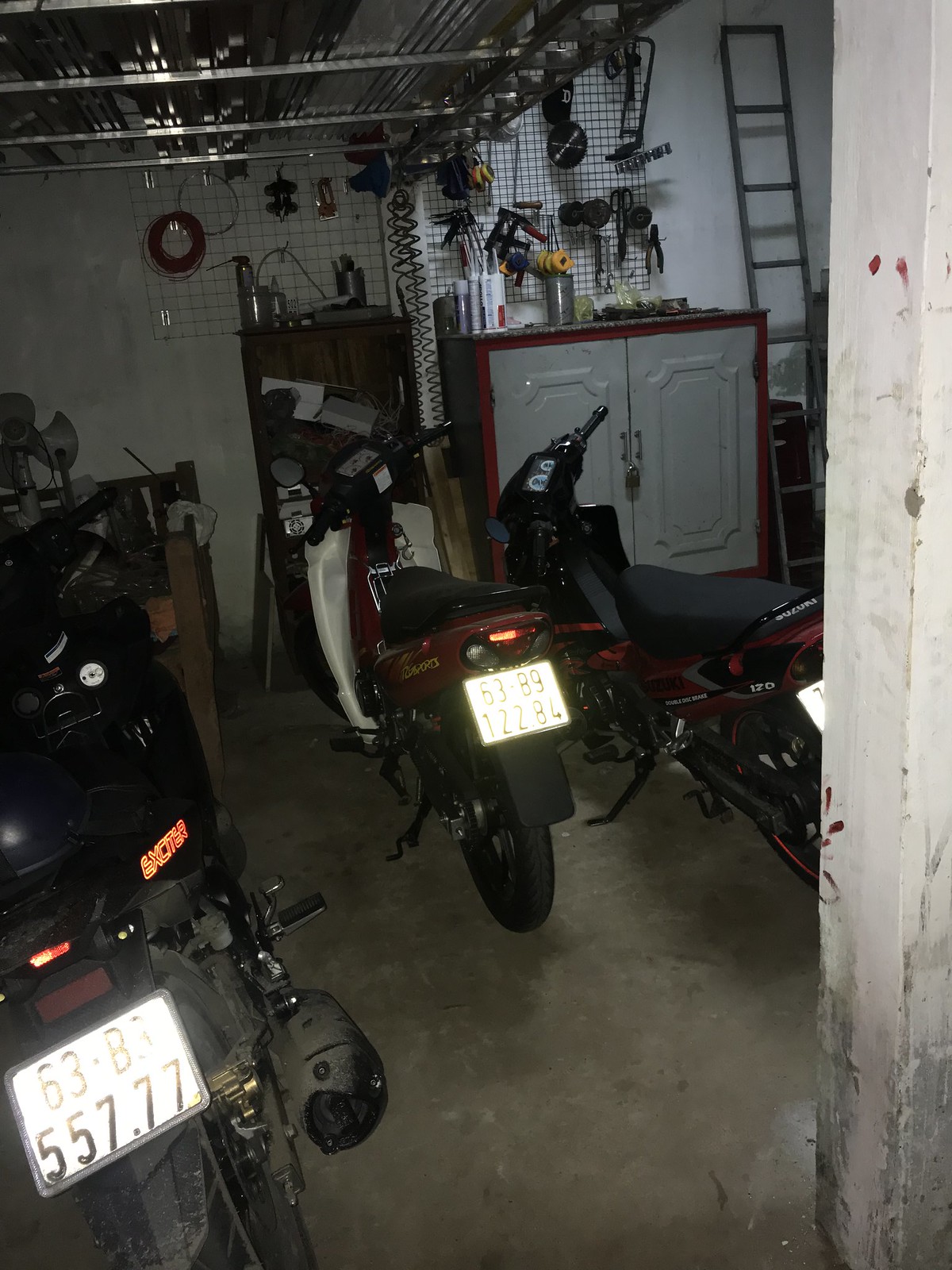The image captures the interior of a garage featuring three two-wheeled vehicles, likely motorcycles or scooters, each adorned with license plates displaying numbers and letters. The middle and right vehicles exhibit black seats with reddish hues, while the left one is entirely black. A white cabinet framed in brown hangs on the wall, flanked by an array of tools organized on a rack. Further to the right, an ascending ladder reaches towards a ceiling storage rack stretching from left to center. A structural post runs along the right-hand edge of the image, supporting the garage's ceiling. The detailed setup underscores a space well-used for vehicle maintenance and storage.